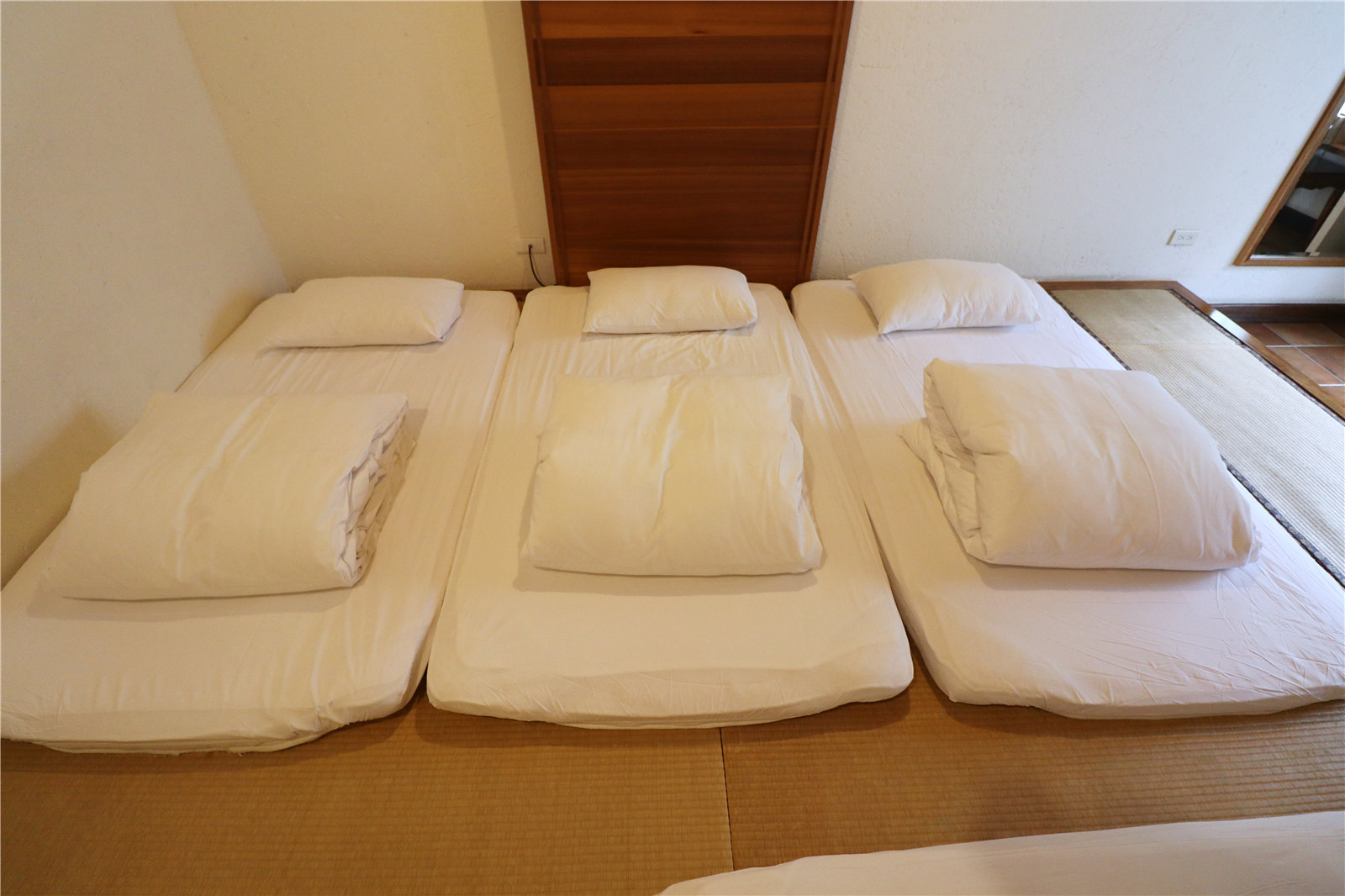The image depicts a room in a Japanese house, possibly in an attic, as evidenced by the sloped, white walls and the general layout. The floor is covered with several tatami mats pushed together, creating a brown surface. On top of the tatami mats are three narrow futons arranged side by side. Each futon is equipped with a folded white comforter at the foot and a small white pillow at the head. The walls are plain white, and there is visible wood trimming around the windows on the right side. A brown dresser can also be seen in the background, adding to the sparse but functional decor of the room.